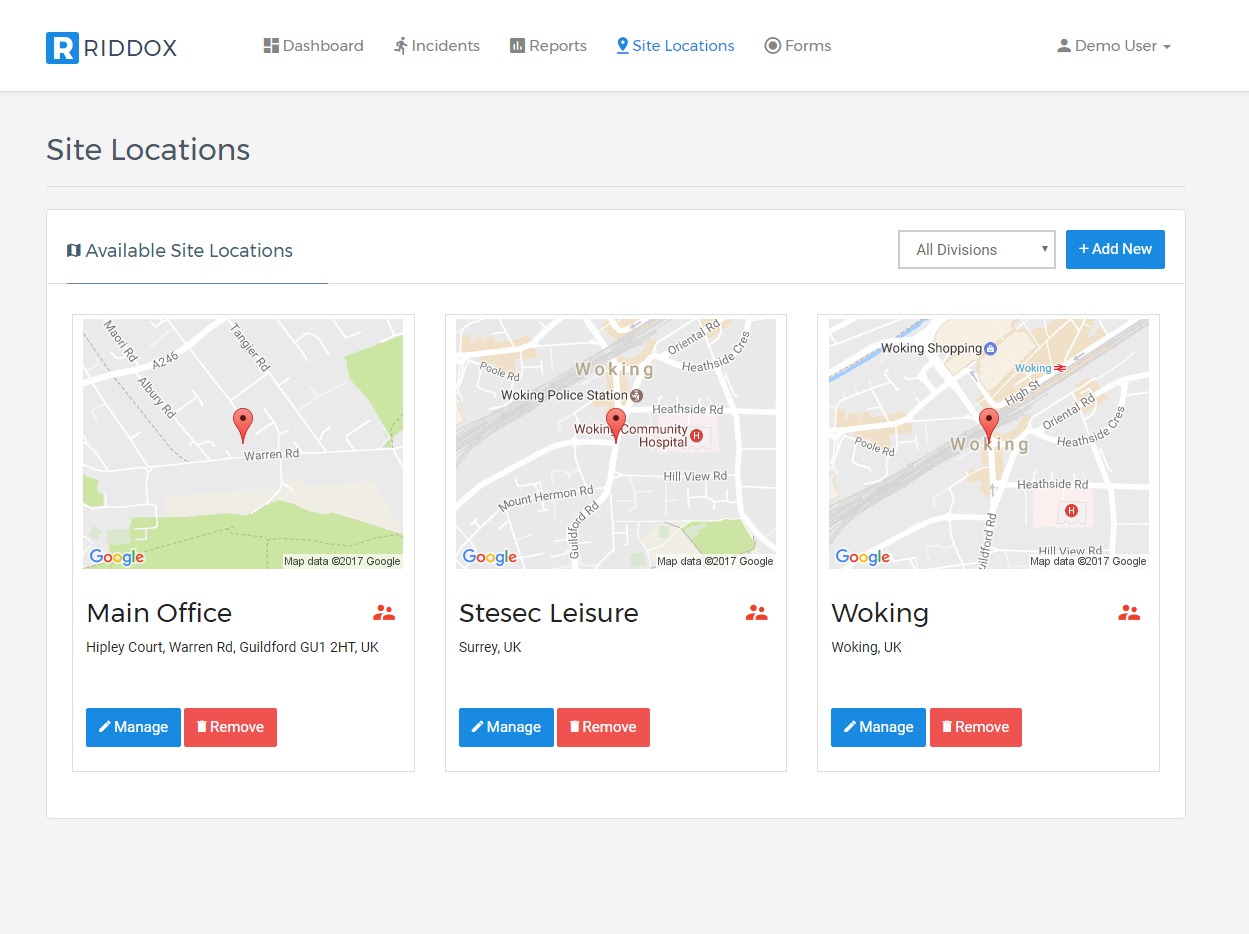The image is a screenshot from a website displayed against a white backdrop. In the upper right-hand corner, a blue box with a red capital "R" inside is present. Next to it, the word "RIDDOX" is written in black letters. Adjacent to this is an icon resembling four pieces forming a box, followed by the label "Dashboard" in black. The subsequent icon depicts a person walking, with "Incidents" written in black text next to it. Moving further, there's a black box labeled "Reports."

Continuing along, there's a blue icon resembling a map pin, with "Site Locations" written in blue. Next to this is an icon of a gray circle outlined by another gray circle, accompanied by the word "Forms." To the right of all this, an icon of a person is followed by the label "Demo User."

Beneath these elements, in bold black letters, the phrase "Site Locations" is displayed. Underneath this heading is a blue and white pop-up bar, where the top left corner contains the text "Available Site Locations" in black, underlined by a black line. To the right of this is a search bar with the placeholder text "All Divisions" in black. Adjacent to it, a blue bar with a white plus symbol includes the text "Add Now."

Below the pop-up bar, there are three separate boxes, each featuring a map image at the top and descriptive text in black beneath. The first box is labeled "Main Office," with further details "Hippley Court, Warren Road, Guilford DU1 2HT, UK." The second box reads "Stasek Leisure" and "Surrey, UK." The third box is labeled "Woking" and provides the details "Woking, UK." At the bottom of each box, a blue box on the left with white text says "Manage," and a red box on the right with white text says "Remove."